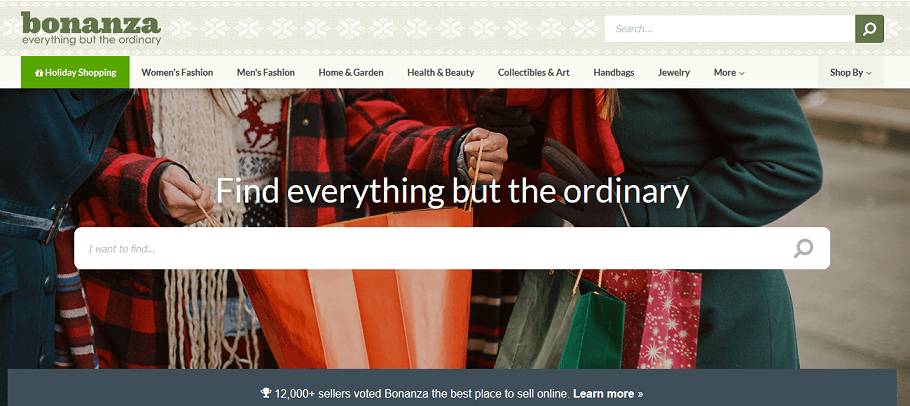**Bonanza Home Page Screenshot Description**

This screenshot features the main or home page of the Bonanza website. The page has a light green design with a white floral pattern that subtly blends into the background. At the top, in bold, dark green lowercase letters, the word "bonanza" is prominently displayed. Beneath this, in smaller text, also in lowercase, is the tagline "everything but the ordinary."

Directly underneath the tagline, there’s a navigation menu consisting of several categories. From left to right, the categories include:

1. **Holiday Shopping** (highlighted in green with white text, indicating it is currently selected)
2. **Women's Fashion**
3. **Men's Fashion**
4. **Home and Garden**
5. **Health and Beauty**
6. **Collectibles and Art**
7. **Handbags**
8. **Jewelry**
9. **More** (indicated by a down arrow suggesting additional options)

To the right of the main navigation menu, there is a light gray button labeled "Shop by" in black text, likely serving as a filter for browsing.

Underneath the navigation bar, there’s a prominent image featuring festive holiday gift bags and people dressed in winter attire. One individual, dressed in a red and black checkered "lumberjack" style jacket, is seen opening an orange bag. Next to this person, partially visible, is another person with a hint of blonde hair wearing a red scarf and a long green winter coat. Only the torsos of the individuals are visible in the image, adding to the cozy, holiday atmosphere.